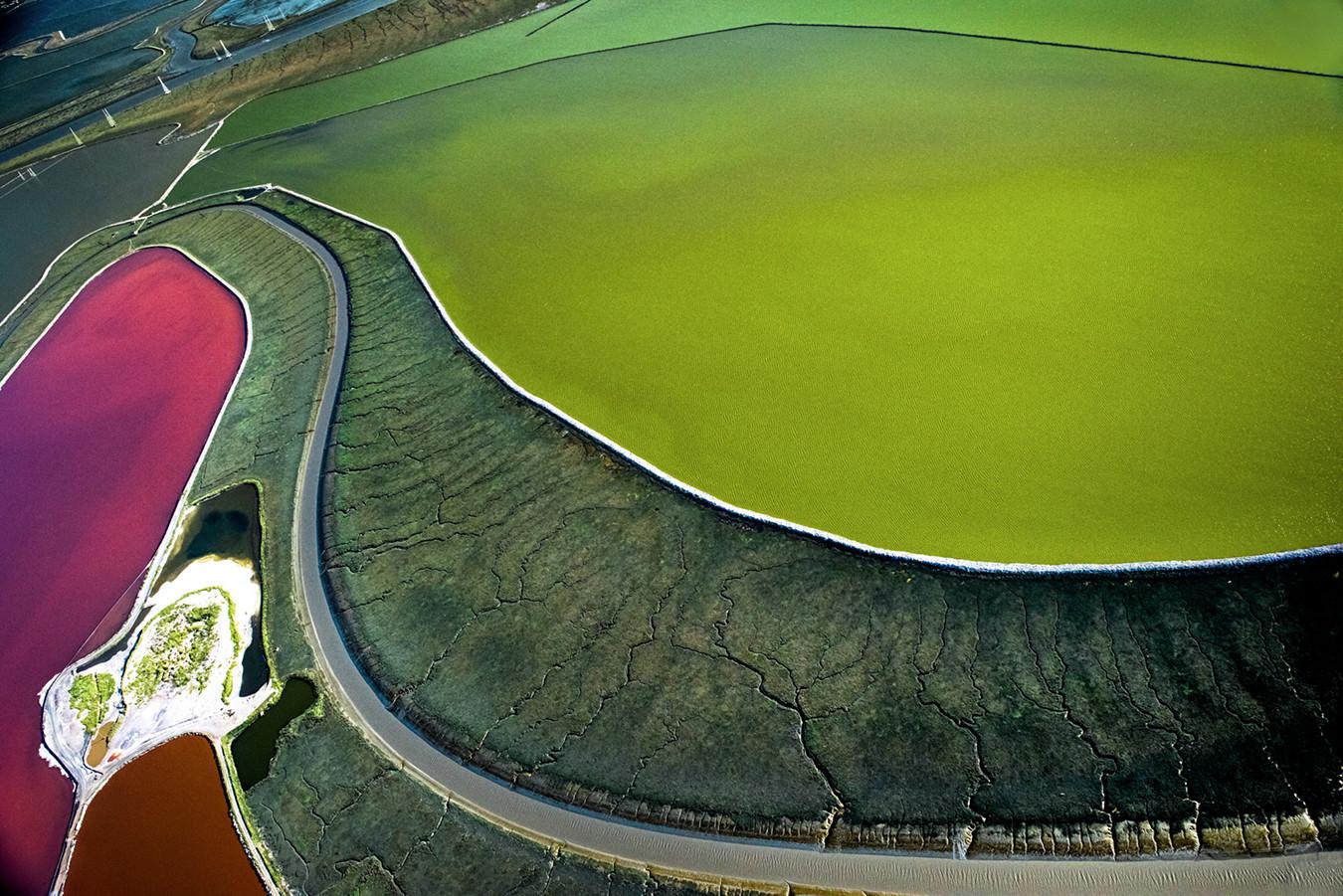This captivating aerial image reveals a vibrant tapestry of varying colors and textures. Dominating the top right quadrant is an expanse of vivid light green, suggesting lush grass or water. A distinctive curving road cuts across the scene from the bottom right to the left, flanked by what appears to be dark, cracked earth, perhaps soil or pavement. A white fence line can be spotted adding a crisp boundary between the green and darker areas. Towards the top left, small, barely noticeable fountains shoot water into the air, adding dynamic movement to the otherwise static scene. Interspersed throughout the left side of the image are intriguing patches of pinkish-purple, contrasting starkly with the earthy colors around it, and a small area of blue suggesting a different body of water. The detailed gradient of green shades complements the occasional brown and white patches, creating a strikingly beautiful and intricate landscape.